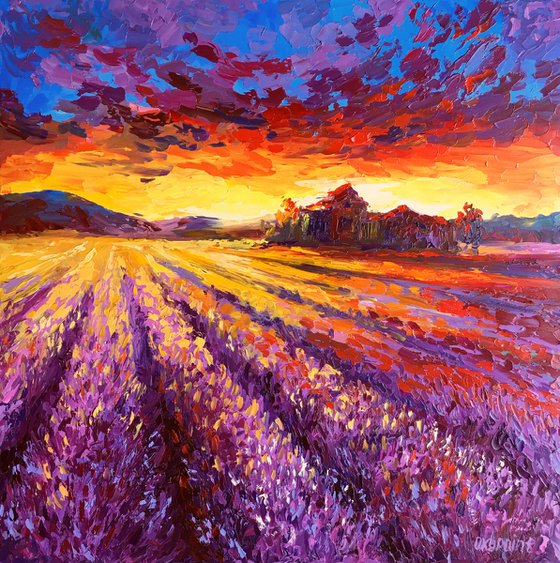The image is a vibrant, impressionistic painting with a blend of watercolors and oil painting techniques. Entitled "A Field of Lavender" by the artist Oxo Point (as indicated by the signature "O-X-Y-P-O-I-N-T" at the bottom right), the scene is an outdoor vista under a striking sky comprised of deep blues, warm oranges, and radiant yellows with hints of maroon and purple. In the forefront, rows of purples and yellows alternate in a mesmerizing lavender field, accented by walking paths in between. These rows are visually wider at the front and narrow toward the horizon, creating a sense of depth. A farmhouse, depicted in hues of orange, gray, and blue, is nestled amid surrounding trees on the right center of the image. Above this, an expressive sky showcases a brilliant yellow sunset, blending with red, purple, and soothing maroon clouds, transitioning into a blue sky. The entire composition evokes a sense of tranquility and timeless beauty, with abstract elements and an overall soft yet vivid color palette that embodies modern impressionism.